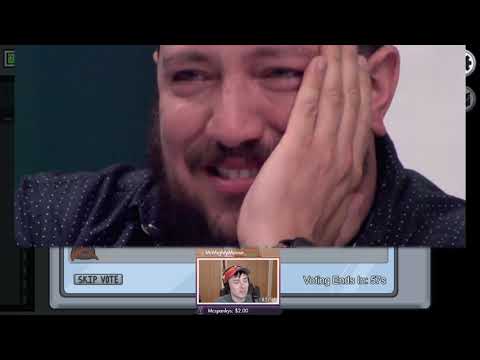The image is a complex composition featuring two overlapping photographs. The dominant foreground photo showcases a gentleman from the show Impractical Jokers, smiling with his right hand covering part of his face. He is looking to the viewer's left and is wearing a dark shirt with very small white dots. His image is set within a rectangle atop another image, creating a layered effect. 

Behind this main image, towards the bottom center, there is a smaller, partially obscured screenshot likely from a livestream or game interface. This lower image features an individual with a red baseball cap, seen speaking into a microphone. Accompanying this smaller image, there are on-screen graphics: the left side reads "skip vote," while the right side includes a button and text that says "voting ends in 50 seconds." Additionally, there's a label beneath the streamer indicating a username and a small donation amount. The background of this lower image is predominantly black with several indistinct elements, making the overall composition visually intricate.